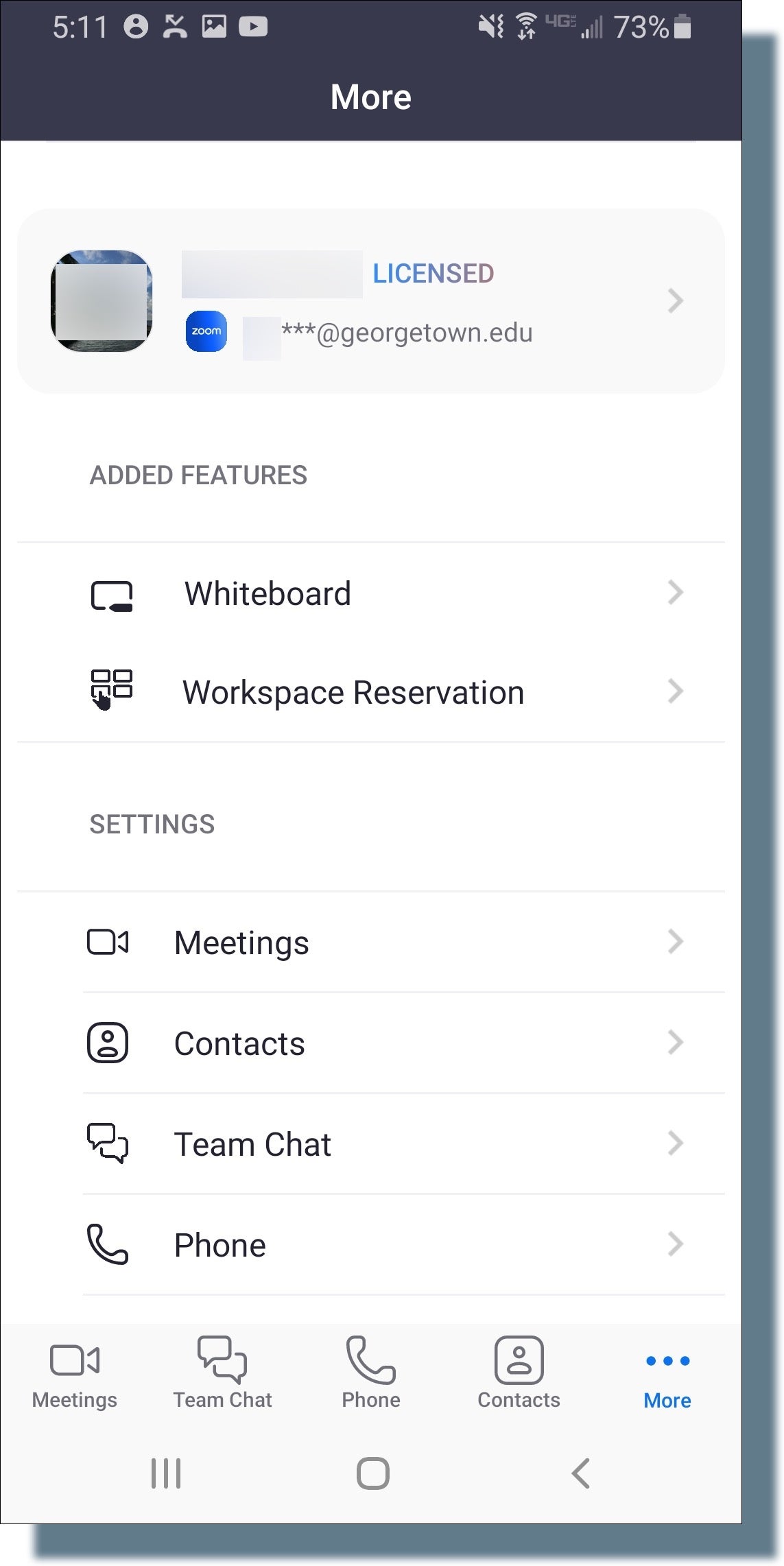The image depicts a smartphone screen with a battery level of 73% and the time showing 5:11. The screen has a strong connection signal. At the top of the page, there's a black header with the word "MORE" in capital letters. The main portion of the screen is white with the word "licensed" prominently displayed in the middle. Beneath "licensed," there is an example from georgetown.edu. Below this, the screen lists several added features. 

To the right, there are clickable icons including a whiteboard image labeled "Whiteboard," and an image of a workspace labeled "Workspace Reservation." Each of these icons allows further interaction. Below these icons, there are more features including "Settings," "Meetings," "Contacts," "Team Chat," and "Phone." The "Phone" feature is represented by a phone icon, "Team Chat" has messenger icons, "Contacts" includes a person icon, and "Meetings" is represented by a box with an extension that resembles a megaphone.

At the bottom of the screen, there is a navigation bar with options for "Meetings," "Team Chat," "Phone," and "Contacts," along with a "More" button highlighted in blue. The blue "More" button indicates additional information and options are available when clicked.